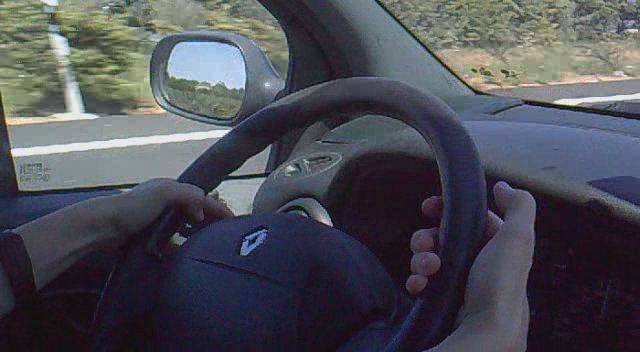This photograph captures an intimate, dynamic moment within a moving car, focusing on the hands of the driver gripping the steering wheel. The image shows the steering wheel from an interior perspective, with one hand positioned at 9 o'clock and the other at 2 o'clock. Part of the windshield, driver's side window, and side mirror are visible, all contributing to the sense of motion suggested by the blurred greenery and trees outside. The hands, the only visible part of the driver, are angled in a way that suggests the photograph was taken from the passenger seat. The steering wheel features an unidentifiable symbol, likely a logo, but no text appears in the frame. The scene effectively conveys the experience of driving through its detailed composition and the subtle suggestion of motion.